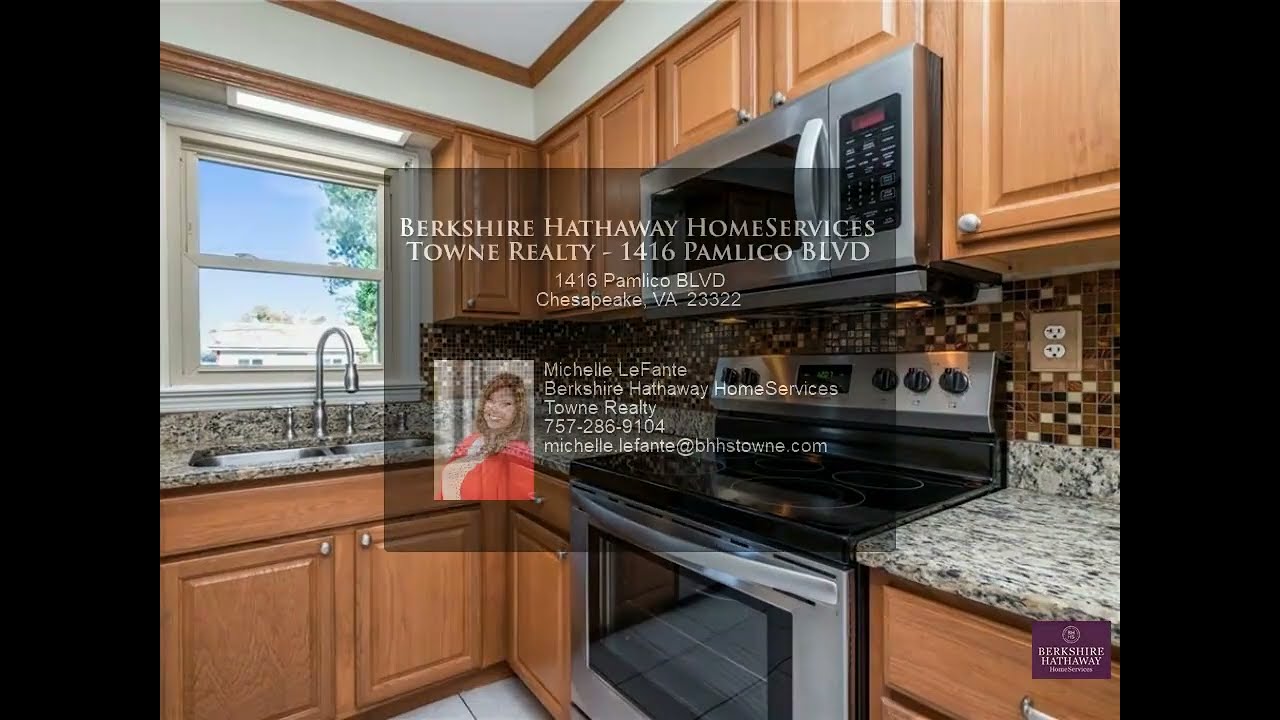The photograph depicts a well-lit kitchen with brown cabinets and gray marble countertops. On the left side of the room, a sink is installed below an open window, offering a view of a blue sky, trees, and an adjacent house. Below the window, a couple of cabinets are visible. On the right-hand side, there is a microwave built into the overhead cabinets that span the wall from left to right. Below the microwave is a combination stove and oven, both featuring stainless steel and black finishes. Adjacent to the stove, there are additional cupboards on the left and drawers on the right.

Occupying the center of the image is a semi-transparent, black rectangular overlay resembling a business card. Across the top, it prominently displays "Berkshire Hathaway Home Services, Town Realty," followed by an address: "1416 Pamilko Blvd, Chesapeake, Virginia, 23322." Below, in capital letters, is the name "Michelle LeFontaine," who is presumably the realtor, along with her contact information including a phone number and email address. To the lower left of the black overlay is a small photograph of Michelle, dressed in a red jacket, reinforcing her role as the point of contact for this property.